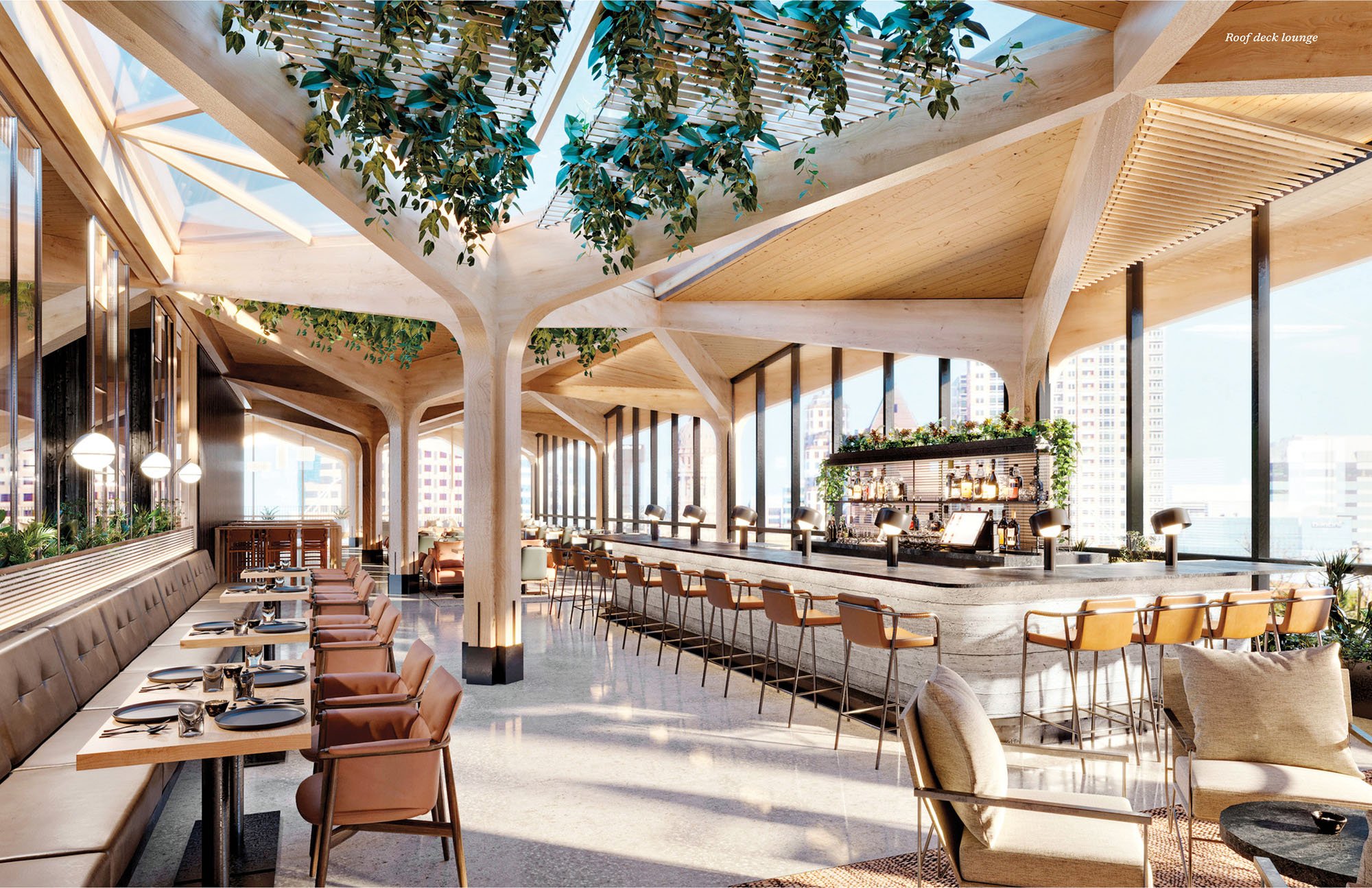This image captures the interior of an expansive rooftop restaurant bathed in sunlight streaming through large, tall glass windows and multiple skylights, creating a bright and airy atmosphere. The seating area to the left features brown leather booths with white cushions, accompanied by light-brown wooden chairs with leather seats arranged around light-colored wooden tables set with black plates, glasses, and silverware. The restaurant's color scheme is predominantly beige, brown, white, and light gray, enhancing its modern, sophisticated look.

In the center, there's a prominent white bar with a sleek black slate top, encircled by orange leather stools with metal legs. Behind the bar, shelves are lined with various bottles of alcohol, and a large computer screen is visible. Small lamps attached to black posts are strategically placed along the bar, casting targeted light onto the counter. 

The ceiling is an architectural marvel, featuring geometric patterns with numerous skylights, some of which host hanging plants that add a touch of greenery to the space. The ceiling is constructed from large wooden beams forming arches that gracefully descend into pillars scattered throughout the restaurant.

On the left-hand side of the image, near the booths, there are several rectangular tables with light-colored wood surfaces. On the right side, you can see some round tables with cream-colored cushioned chairs arranged around them. The space appears meticulously prepared for the upcoming lunchtime rush, with all tables set and waiting for patrons.

A subtle white label in the top right corner reads "Roof Deck Lounge," affirming the restaurant's elevated location atop a skyscraper, offering diners a panoramic view of the surroundings.